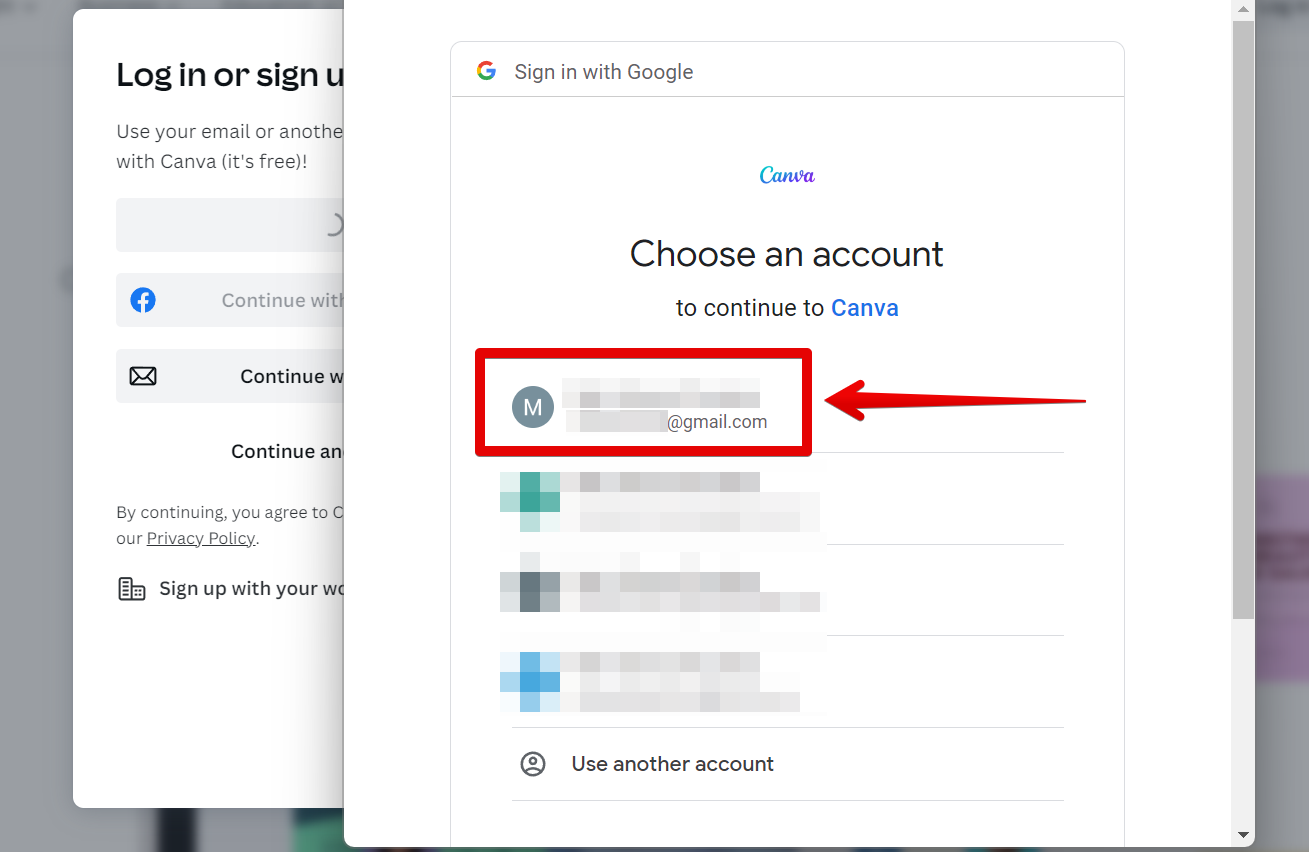The image depicts the sign-in process for Canva using a Google account. In the foreground, a pop-up window prominently titled "Sign in with Google" is displayed. Below this title, the text "Choose an account to continue to Canva" is visible. The pop-up features a gray circular icon with the letter "M" in the center. Some text is blurred, but a specific email address ending in "@gmail.com" is highlighted with a red rectangle and an arrow pointing towards it, drawing attention to the selected account.

Beneath the primary account, there are three more blurred options for signing in, as well as the option to "Use another account." 

In the background, there are two noticeable layers. The first layer, covered with a gray filter, displays the main Canva login or sign-up page. Over this, a second white layer appears, giving context to the pop-up window, indicating the user is at the Canva login screen, which is free to access. 

The color scheme includes shades of gray from the background filter, white from the pop-up and login layers, and additional colors such as black, blue, red, yellow, green, and purple, detailing various elements of the interface.